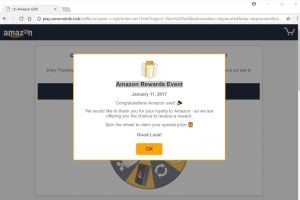This image, with dimensions of 300x200 pixels and a file size of only 9 kilobytes, is an extremely small and blurry screenshot. It depicts a desktop view of a website, though it is challenging to identify the specific browser or operating system in use. In the address bar, a long, complex URL is visible, starting with the word "play" but too pixelated to decipher further. The top left corner of the website displays the Amazon logo, while the top right features an icon of a shopping cart. However, despite these familiar elements, this is evidently not an actual Amazon website.

Superimposed on the site is a pop-up featuring a white and yellow gift box, emblazoned with the text, "Amazon Rewards Event, January 11th," presumably from the year 2017. The message continues with "congratulations" followed by illegible text, and ends with an invitation to try your luck and two buttons, likely "OK" and another unclear option. Behind the pop-up, there appears to be a spinning wheel, suggesting a game to win various prizes.

Overall, the image is a classic example of a scam, attempting to deceive viewers into believing they've won an Amazon gift card. This fraudulent pop-up is a stark reminder to remain cautious of unsolicited reward notifications online.